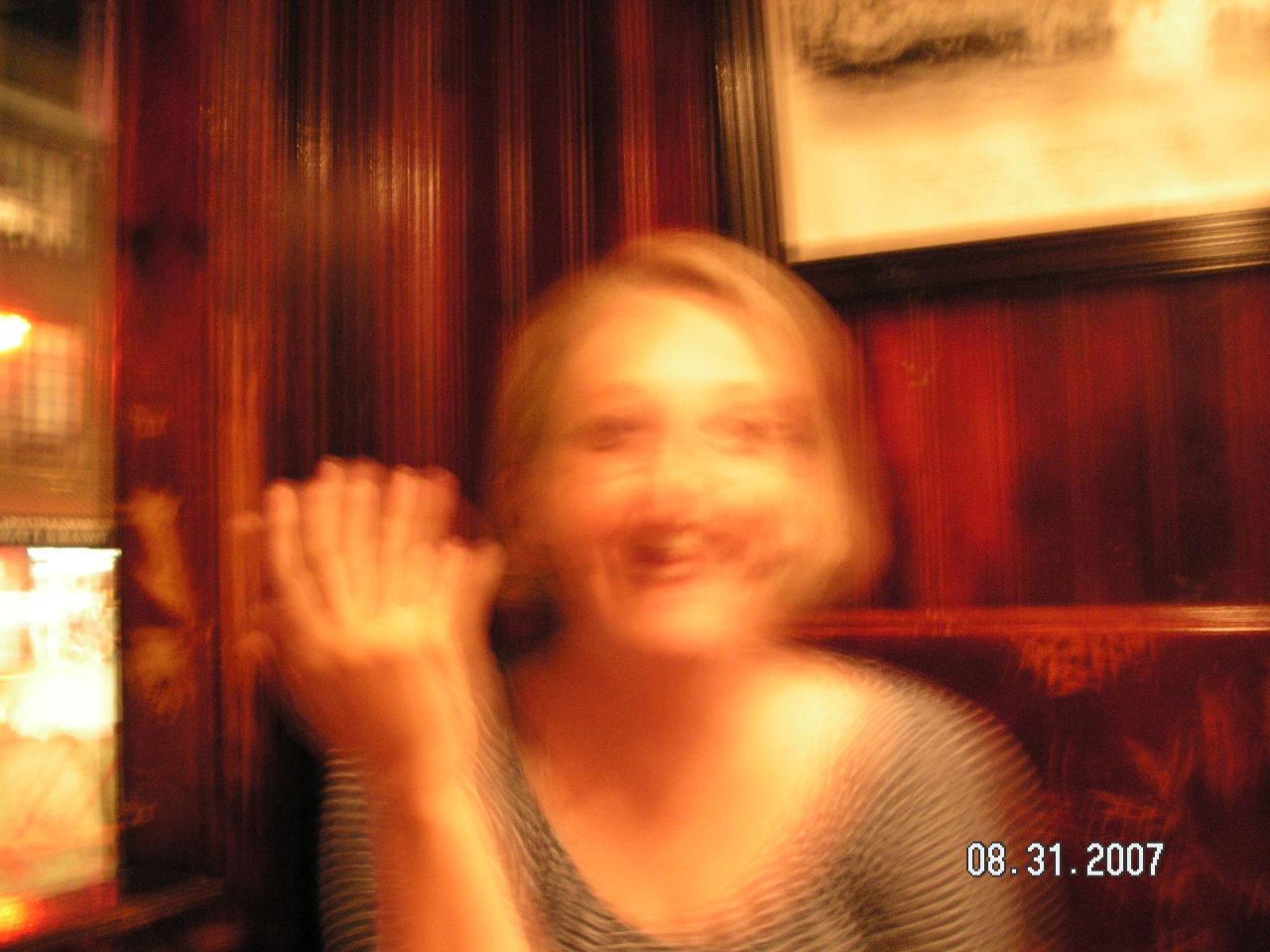In this photograph, a young woman is seated in a restaurant booth, flashing a warm smile despite the image's noticeable blur and lack of focus. Her just-short-of-shoulder-length blonde hair frames her face, and she is wearing a low-cut black and white striped top. One of her hands is raised to the side, where motion blur creates the illusion of multiple fingers. The background features a rich, cherry wood-colored wall and booth seating adorned with a light floral design. Sunlight filters through a window on the left, partially obscured by a gray shade. A black-framed piece of wall art with a tan canvas adds a touch of decor. A date stamp on the bottom right corner reads "08.31.2007," marking this moment in time.